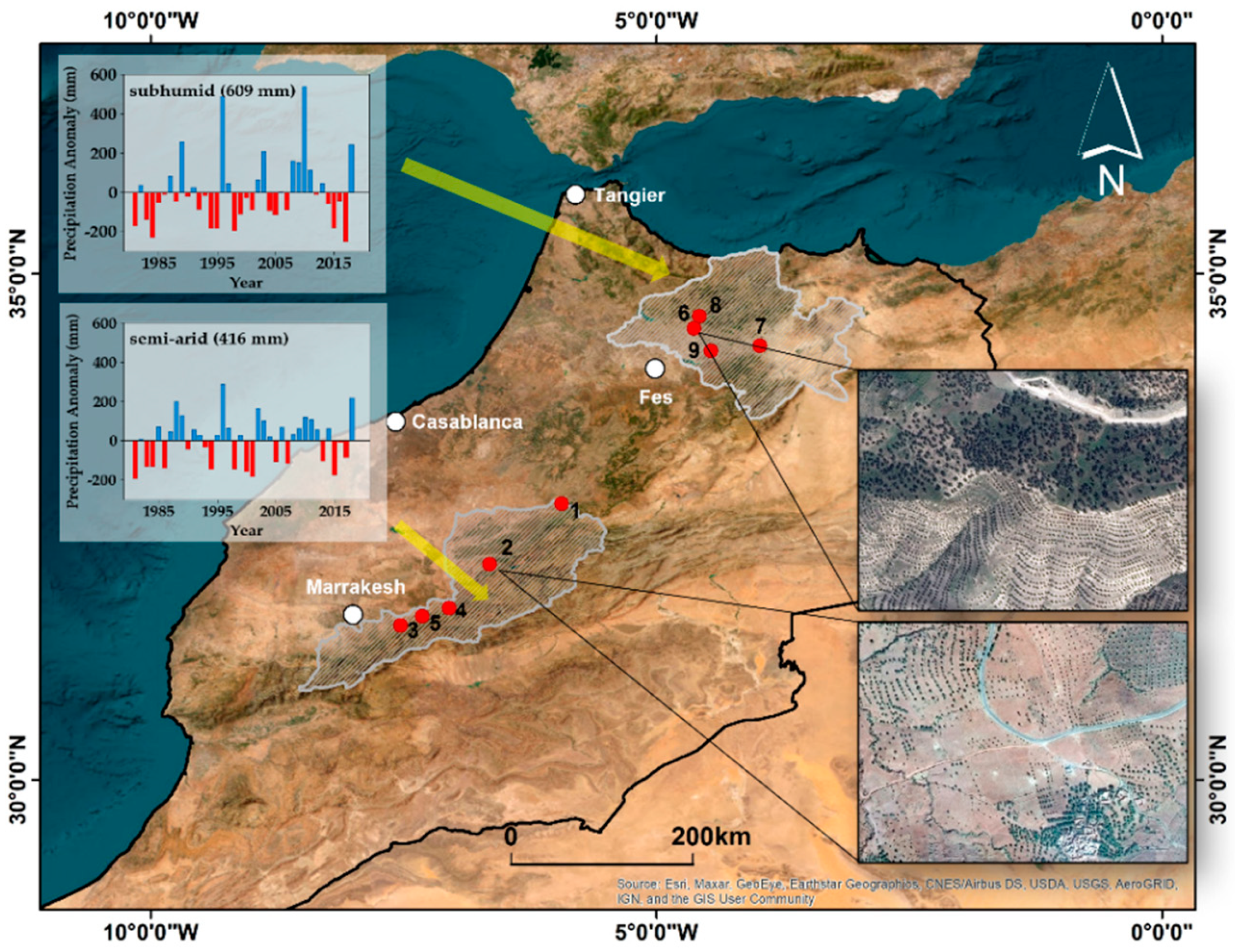The image is a detailed map of northern Africa, featuring several infographics and topographical insets. In the upper left-hand corner, there are two precipitation anomaly graphs labeled "sub-humid" (609 mm) and "semi-arid" (416 mm). These graphs, each with an x-axis representing years and a y-axis representing precipitation anomalies, show bars in green and red indicating variations in annual precipitation.

The main map highlights various geographical landmarks and bodies of water, including an ocean on the left side and an inlet or gulf in the central portion. A large landmass extends from the upper right to the bottom left of the image, with smaller landmasses visible in the north. Key cities such as Marrakesh, Casablanca, and Tangier are marked on this map.

On the right-hand side of the image are two zoomed-in topographical maps, displayed in rectangles. These insets provide aerial views of certain regions highlighted by red dots and numbers on the main map. The topographical overlays correspond to specific areas marked in gray on the main map, with labels ranging from 1 to 9, showcasing different landforms and conditions.

Overall, the image combines cartographic and graphical data to provide a comprehensive visualization of northern Africa's topography and precipitation patterns.